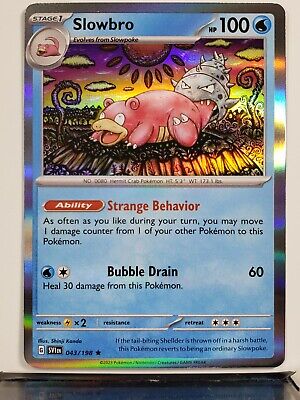This is a Pokémon trading card, enlarged into a poster, displayed on a white background wall with a dark table or possibly a black line running underneath it. The card, which is typical trading card size, prominently features Slowbro, a large, pink, hippopotamus or bear-like creature illustrated in an anime style. Slowbro has a yellow beak and yellow lines on its belly, and from behind, a large, silver, fish-like creature is biting its tail. The background behind Slowbro is a vibrant mix of yellow, red, and purple, with yellowish-white clouds in the sky, and multicolored boards underneath him.

In the upper left corner of the card, "Slowbro" is written, while the upper right corner denotes its HP as 100. Below the illustration, there is a red text description of Slowbro's ability called "Strange Behavior," which states: "As often as you like during your turn, you may move one damage counter from one of your other Pokémon to this Pokémon." Below this ability, it also mentions a move, "Bubble Drain 60." Additional game details, such as experience points and other statistics, are marked by dual white lines at the bottom. The card also notes that Slowbro is a Stage 1 Pokémon, which evolves from Slowpoke, indicating its progression in the game.